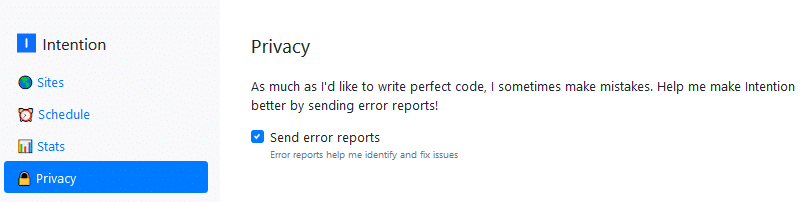The image is a simple screenshot with a white background. On the left side, there is a gray vertical rectangle divided into five sections. 

1. At the top of the gray rectangle, in black font, it says "Intention." To the left of "Intention" is a blue square containing a white eye icon.
2. Below "Intention," the second section has the word "Sites" in blue font with a globe icon to its left.
3. The third section contains the word "Schedule" in blue font with an alarm clock icon to its left.
4. The fourth section says "Stats" in blue font, accompanied by a small bar graph icon on its left.
5. The fifth and bottom section, "Privacy," is written in blue font with a padlock icon to its left. This section is highlighted with a blue rectangle, indicating it has been selected.

On the right side, against the white background, the word "Privacy" appears in black font followed by the text: "As much as I'd like to write perfect code, I sometimes make mistakes. Help me make my intention better by sending error reports." 

Below this text, there is a blue checkbox with a white checkmark in it. Next to the checkbox are the words "Send Error Reports" followed by a sentence in smaller font: "Error reports help me identify and fix issues."